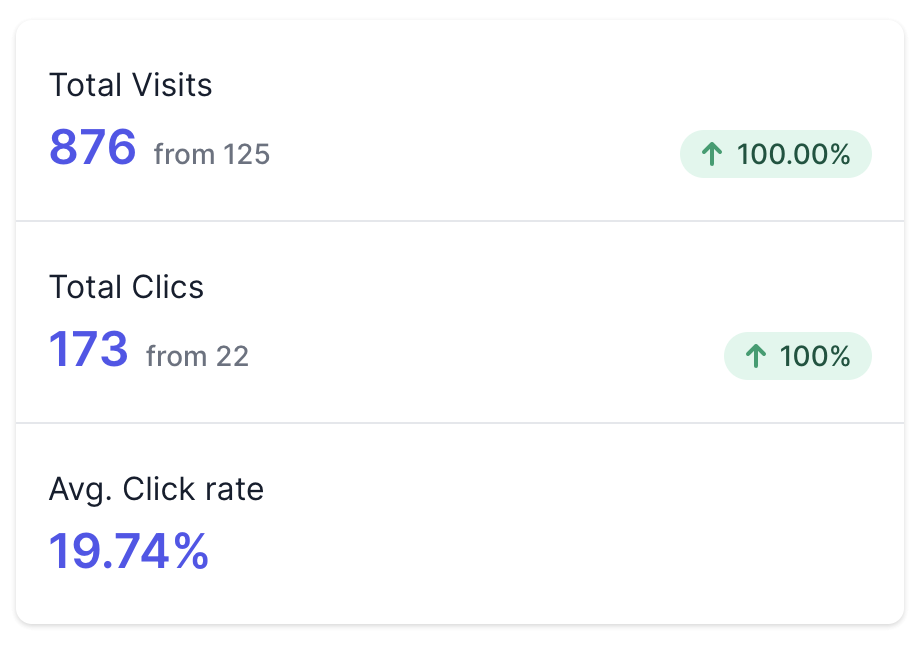This digital screenshot depicts various metrics related to website activity. 

At the top, the section labeled "Total Visits" showcases a bold, purple number "876," indicating the total number of visits. Adjacent to this, a green button with an upward-pointing arrow displays a "100%" increase.

Beneath this, the "Total Clicks" section features a bold, purple number "173". To the right of this figure, another green button with an upward-pointing arrow indicates a "100%" increase.

Further down, there is a section labeled "Average Click Rate," abbreviated as "AVG." in black font. The associated metric, shown in bold purple, is "19.74%".